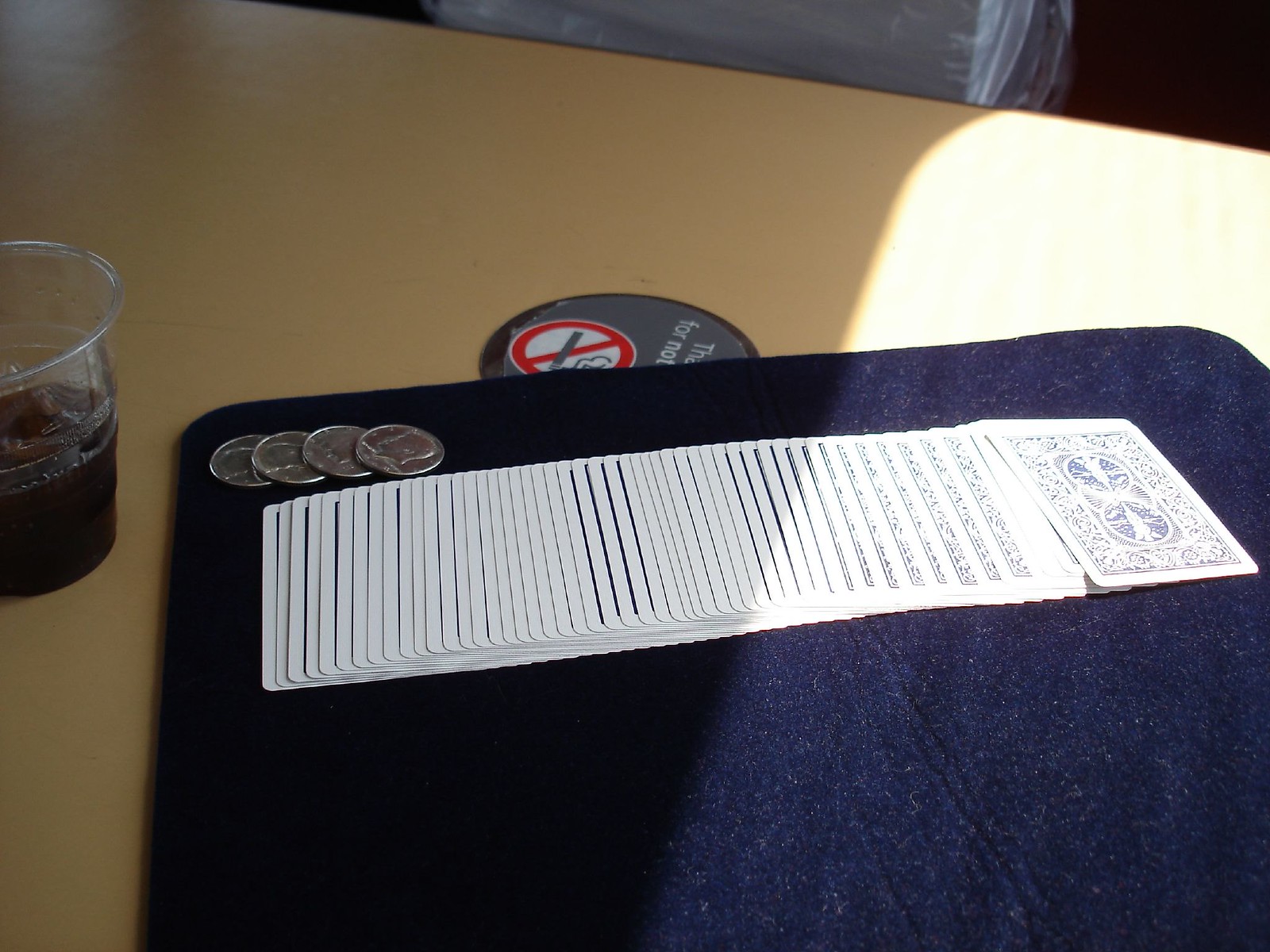The image depicts a casual scene centered around a table, which is more wide horizontally than it is vertically, resembling a horizontal rectangle. Although the picture appears to be taken with an iPhone or a budget digital camera, it captures the setting with reasonable clarity. 

The focal point of the image is a table with a prominent "No Smoking" sign placed in the middle. Draped over the central area of the table is a plush, blue velvet placemat. Arranged horizontally across the placemat is a deck of playing cards, all turned face down, showing only their patterned backs. 

On the top left corner of the placemat, a small stack of four quarters is scattered, with some coins slightly overlapping each other. Adjacent to this tableau, on the left side of the table, stands a clear plastic cup filled with a dark brown liquid, suggesting it could be either cola or a type of alcoholic beverage.